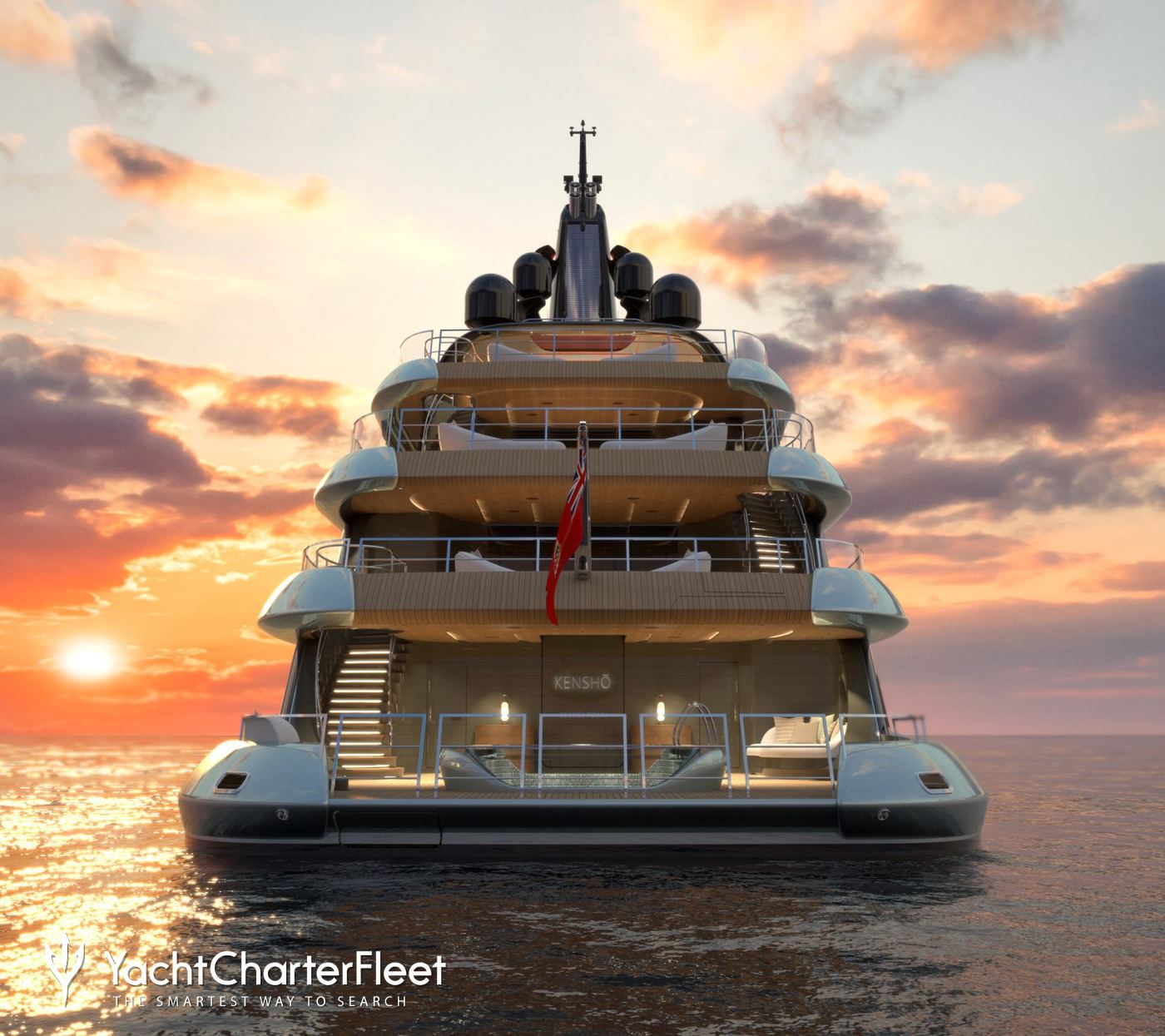In this professionally taken photograph, the majestic white yacht, named Kensho, dominates the center with its impressive four levels, each featuring distinct details. On the lower deck, chairs are neatly arrayed alongside a gracefully sweeping stairway leading to the second deck. The upper levels reveal more seating arrangements, while the very top deck captures a unique scene: two men bowing, facing another man holding a religious item aloft, suggesting a ceremonial moment. The yacht itself is set against the serene backdrop of a sunset, with hues of orange, purple, and blue blending seamlessly in the sky, dotted with dark gray, orange, and yellow-tinged clouds. The calm ocean reflects the sparkling twilight as the vessel sails forward. In the lower left corner, a logo featuring a Y with a line through it and the text "Yacht Charter Fleet, the smartest way to search" marks the image as part of an advertisement or flyer.